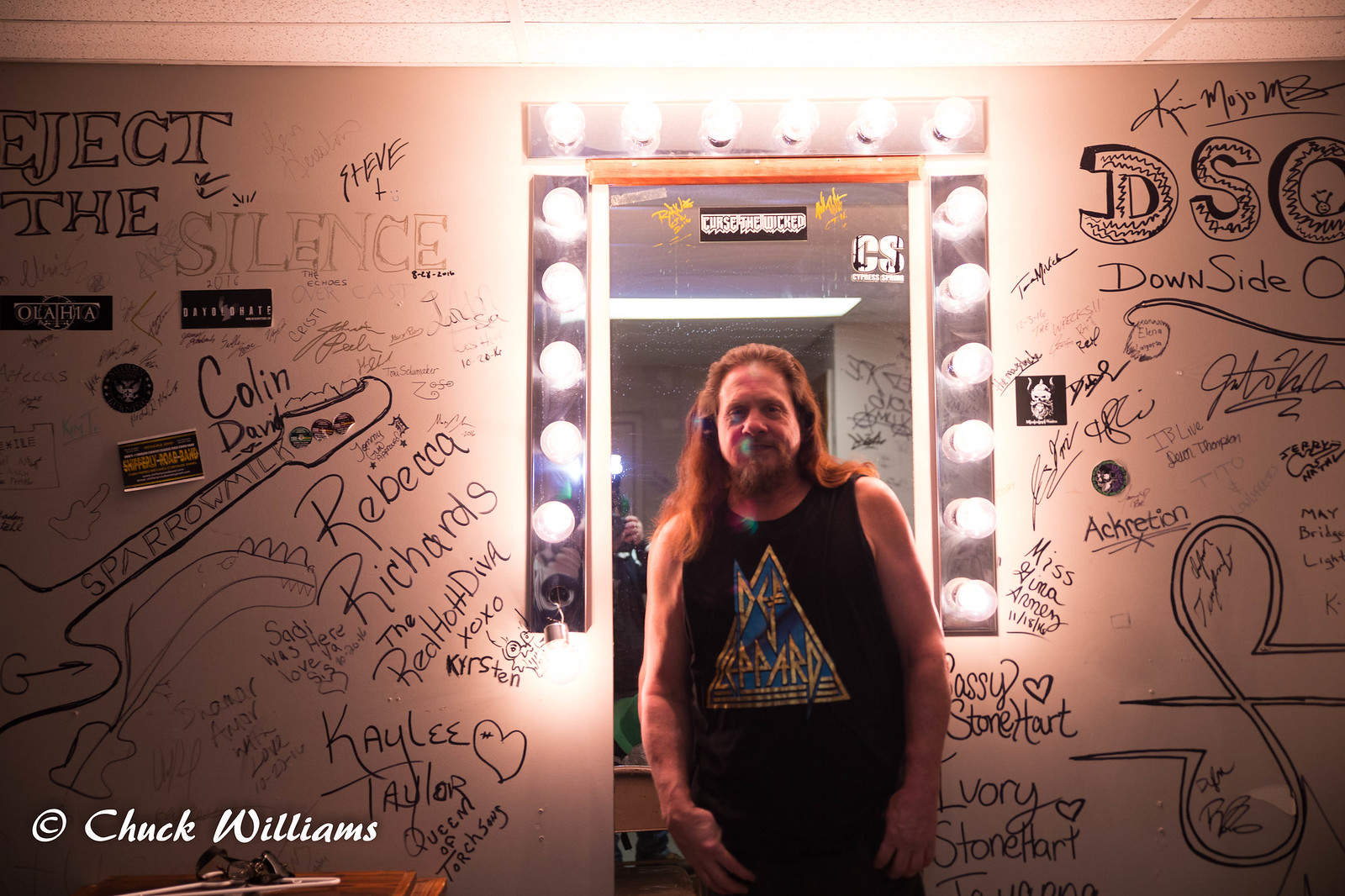In this striking image, a man stands confidently in front of a brightly lit mirror, framed with round light bulbs reminiscent of a backstage dressing room setup. The lights, glowing vividly, encircle the mirror's edges from top to sides, casting a radiant glow. The man's reflection is visible in the lower corner of the mirror, showcasing his long red hair flowing down to his shoulders and a neatly groomed red goatee. He sports a black sleeveless shirt featuring a distinctive blue and gold triangular emblem with "Deaf Leopard" emblazoned across the front. His hands rest by his sides as he faces the viewer.

The white walls behind him are adorned with a chaotic tapestry of handwritten graffiti and signatures in black ink. Prominent among the scribbles are names such as "Rebecca Richards," "The Red Hot Diva," "Steve," "Colin," "David," "Kirsten," "Kaylee," "Taylor," and "Queen of Torch Song Sing." Some phrases stand out, including "reject the," "DCS," "Downside," and "Spiral Milk" written near an outlined guitar drawing.

At the bottom left corner of the picture, the photographer's name, "Chuck Williams," is inscribed in white. Beside it, a circled "C" indicates copyright. The collective signatures, drawings, and eclectic writings give the image a raw, rock-and-roll ambiance, capturing the essence of a moment in a vibrant, graffiti-filled environment.